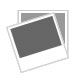The monochrome, black and white image features a rugged Jeep or Land Rover-type vehicle navigating through a watery terrain, with water splashing dramatically around it. The vehicle's windows are rolled up, and its distinct rectangular windshield and grill are prominent. In the background, grainy yet towering pine trees stretch upward, adding to the adventurous ambiance. An inset magnified close-up of a car's headlight sits in the bottom left corner, with water splashing up in a ghostly arc around it. Overlaying a black gradient at the very top of the image, bright mustard-yellow text declares "IP68 waterproof." Below this text are two checkmarks, with the accompanying descriptions "Sealed design protects lights from extreme weather conditions" and "Working temperature, -40°C to -80°C," emphasizing the durability and resilience of the advertised vehicle lights.